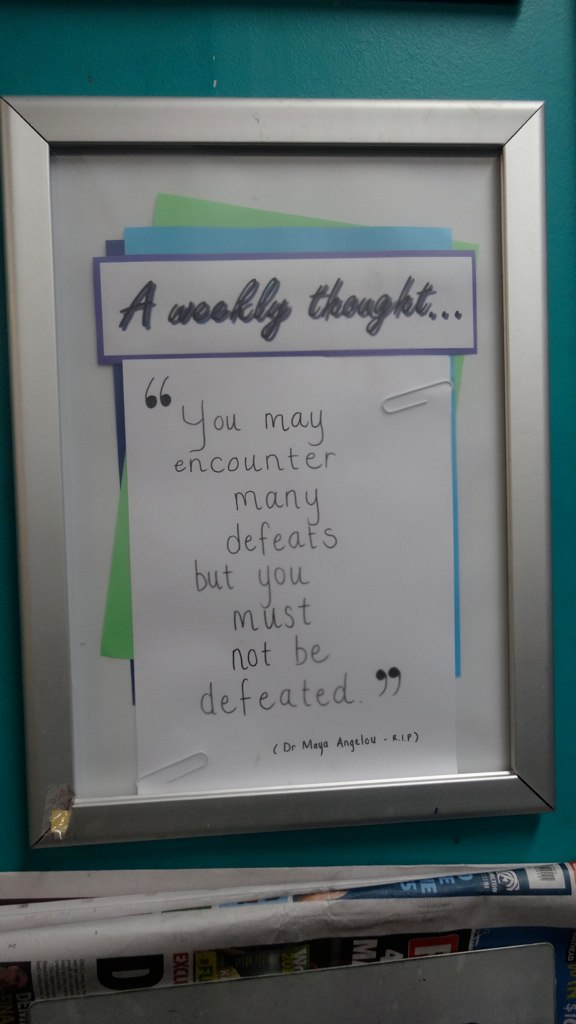The tall rectangular image showcases a framed sign hanging on a wall painted in a deep turquoise color. The frame itself is silver and contains a white background with several overlapping pieces of paper: a dark blue one at the bottom, a neon green one tilted in the middle, and a light blue one on top. Highlighted at the top of the sign is a white rectangle bordered by purple, displaying in cursive the phrase "A weekly thought...". Below this header, the inspiring quote reads: "You may encounter many defeats but you must not be defeated," attributed to Dr. Maya Angelou, with a notation "Dr. Maya Angelou (R.I.P)." The image's lower edge captures the partial view of a newspaper.